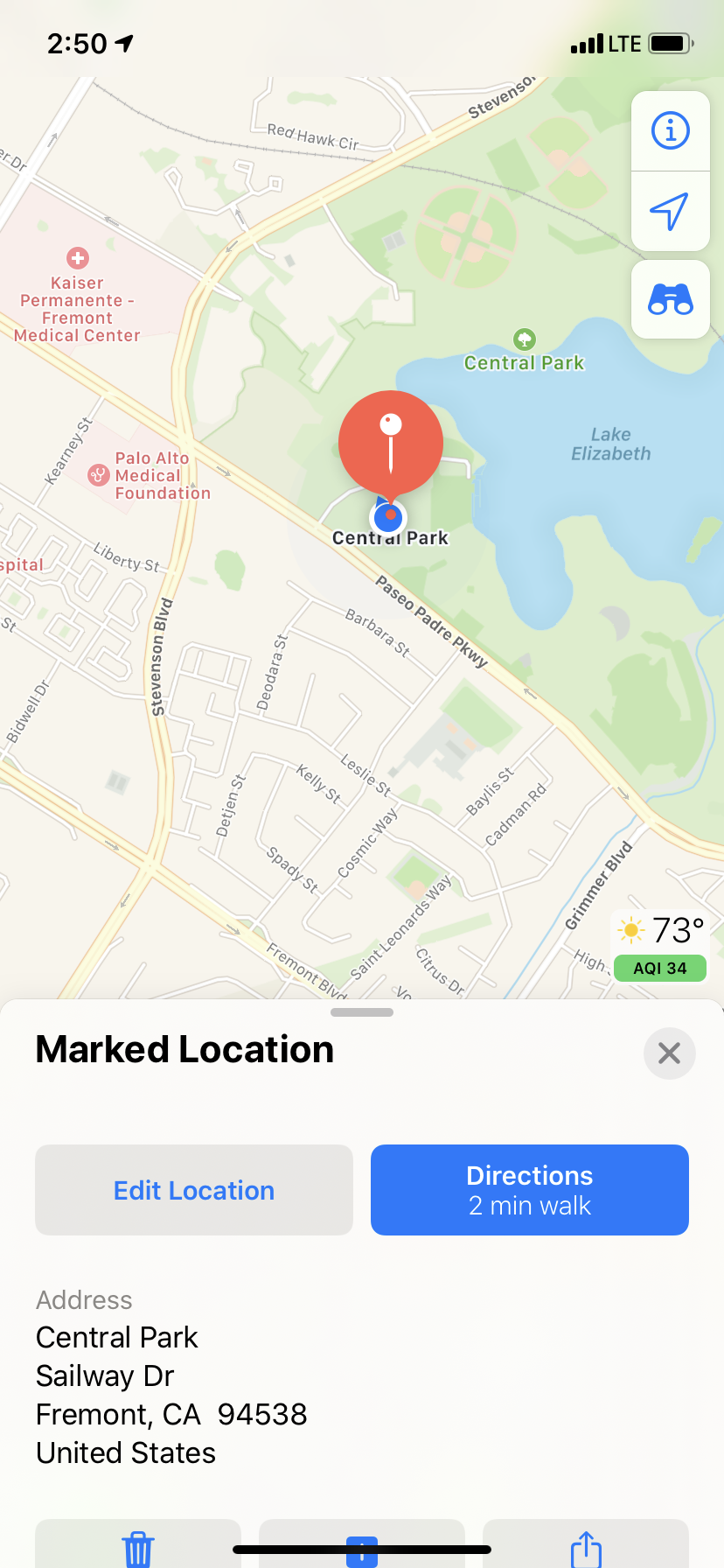This is a comprehensive screenshot from a smartphone mapping or directions application. At the very top of the screenshot, the status bar indicates the current time of 2:50. The device is receiving maximum signal strength with five bars and the battery level is almost full. Centered on the screen, a pin has been dropped on a map, marking a specific location. Surrounding this dropped pin, a large lake and a green space, likely a park, are visible towards the right side of the screenshot. On the left side, various streets and notable businesses or locations are labeled by the app.

Beneath the map, the designation "Marked Location" is displayed. There's a gray button labeled "Edit Location" alongside a blue button that prompts directions, indicating it's just a two-minute walk to the marked location. The full address of the marked location is detailed as "Central Park, Sailway Drive, Fremont, California, 94538, United States." Further below, several action buttons typical of smartphone interfaces are present, including icons for trash (delete), share, and a message or communication option. This intricate map view offers clear navigation and efficient functionality for users seeking directions or additional details.